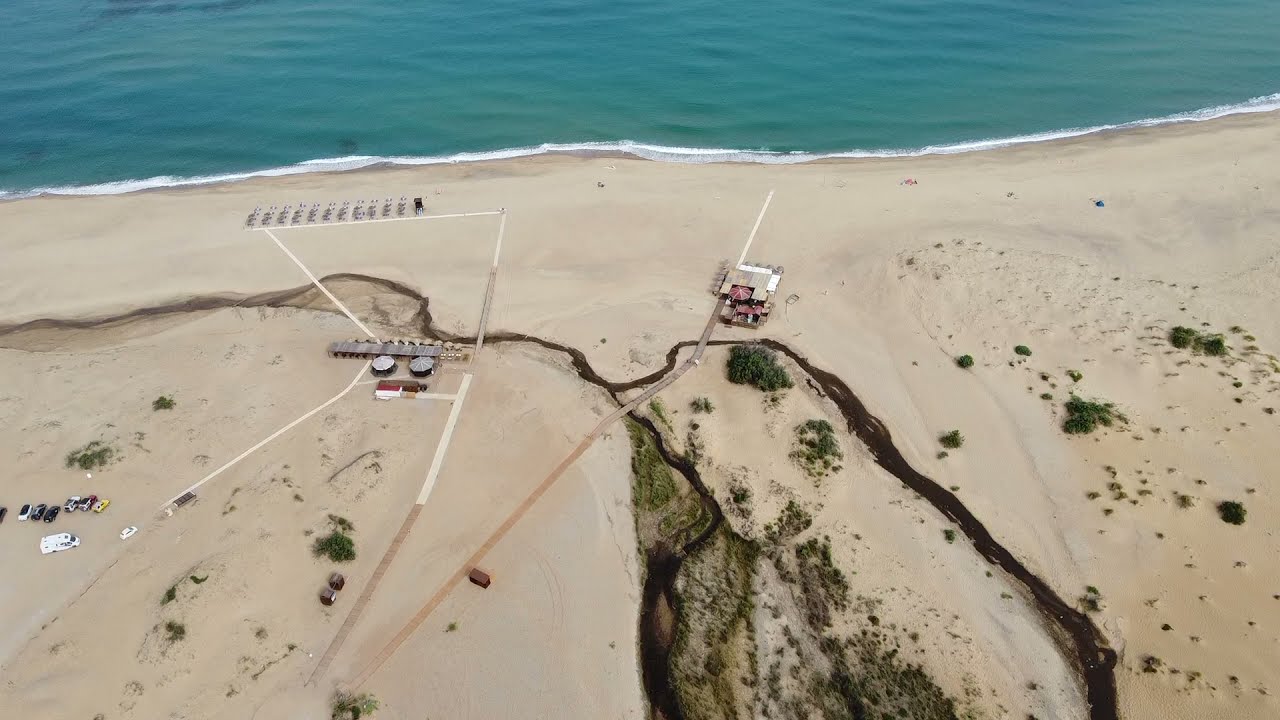This high-resolution, overhead photograph captures a long stretch of a beach adjacent to a blue-green body of water, likely an ocean. The top 20% of the image reveals the water with white, foamy surf crashing against the shore, while the remaining 80% is a sandy expanse. The beige sand dominates the scene, punctuated by patches of green shrubs and bushes. Dark and light-colored pathways crisscross the beach, suggesting boardwalks and access routes.

Central to the image is a wooden or wood-colored house with canopied areas. Extending from this house, various pathways lead towards the water and to a nearby long, thin structure, possibly a restaurant, featuring outdoor patio tables and small adjacent buildings. Near the water’s edge on the left, rows of beach chairs are neatly lined up.

In the bottom-left corner is a noticeable, albeit primitive, parking area in the sandy terrain, with numerous parked vehicles including a recognizable white camper van. The photograph’s wide angle provides a comprehensive view of this tranquil, beachy area making it appear almost serene despite the presence of some industrial-looking buildings.